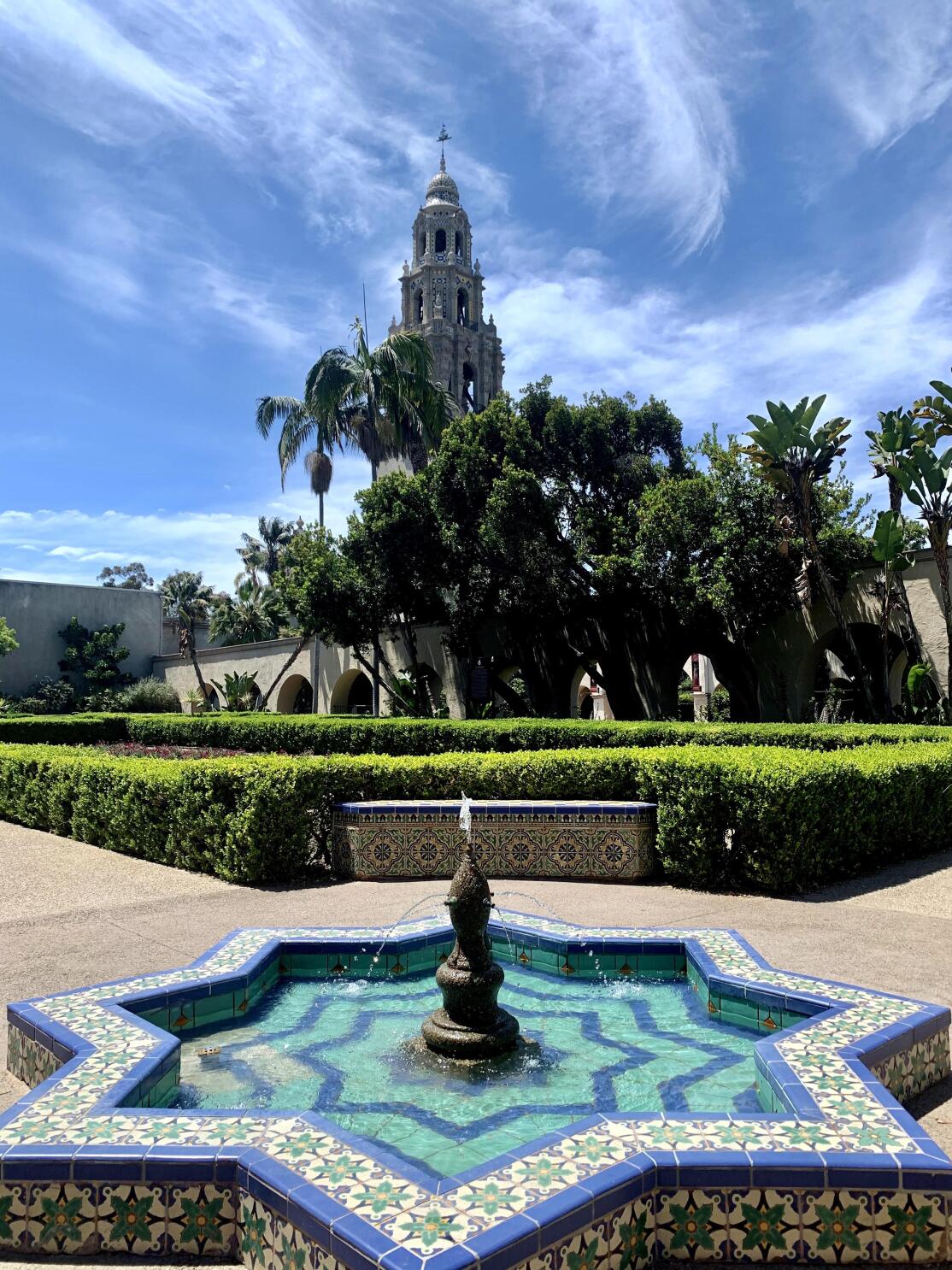This photograph showcases a serene outdoor scene dominated by a seven-pointed, star-shaped fountain, which features green and white star patterns and a blue tile border along its edges. The fountain has water gracefully squirting from a central piece. Surrounding the fountain is a cement pavement and beyond that, a path bordered by precisely manicured, flat, squared-off hedges.

In the mid-ground, there is an intricately designed bench with ornate tile work, set amidst the hedge layout that resembles a maze. Tall, lush trees, including several palm trees, frame the background, creating a verdant backdrop.

Behind the trees stands an impressive, tall structure with a spire or perhaps a steeple that reaches into the sky, suggesting a religious building, possibly a church or synagogue given the faint cross at the top. The photograph is bathed in the natural light of a clear day, with a dark blue sky adorned with wispy white clouds. The scene suggests an idyllic, well-maintained park, potentially hinting at a Middle Eastern location, such as Israel. There are no people or animals visible in the snapshot, enhancing its tranquil and timeless quality.